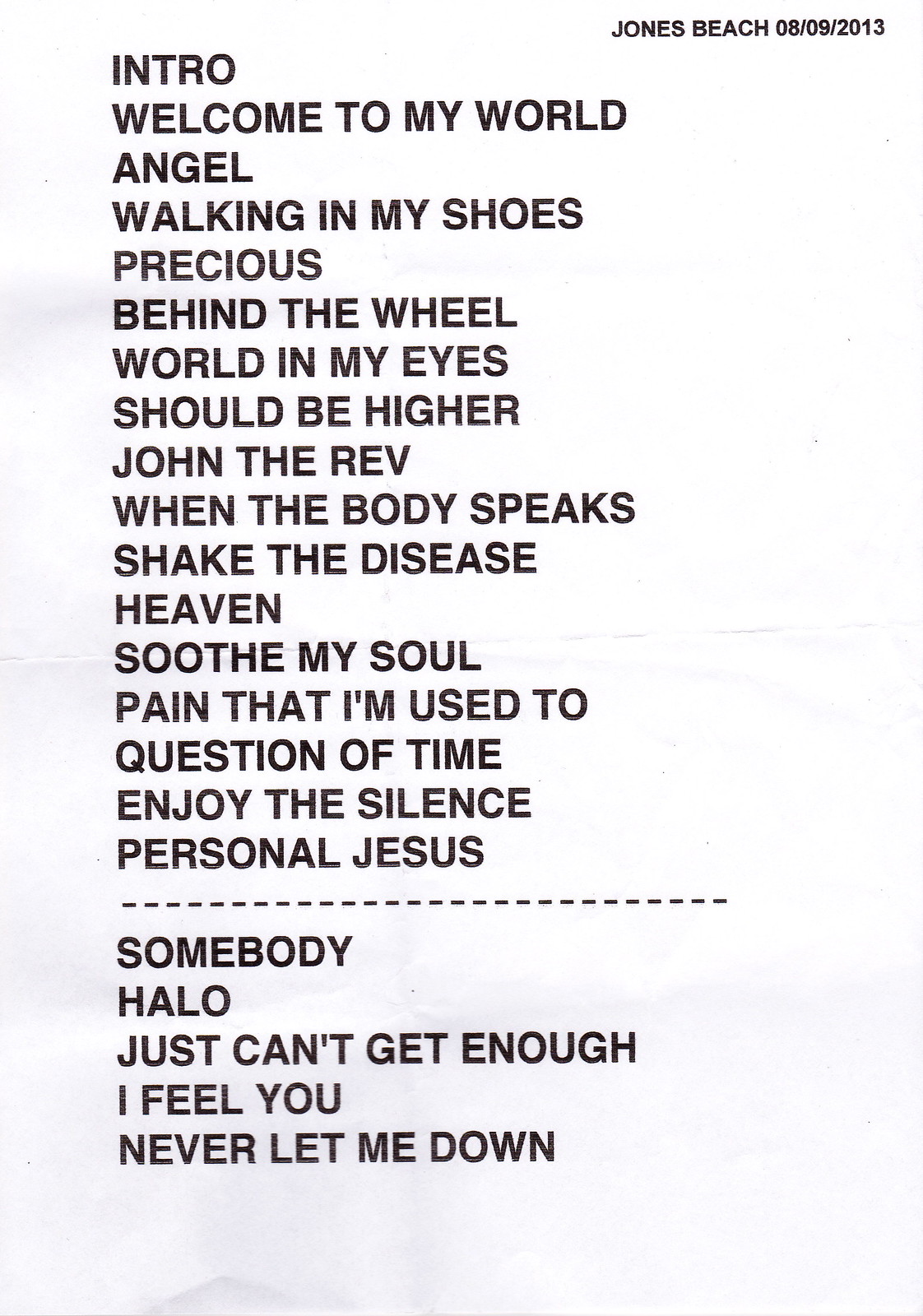The image displays a structured list, possibly of songs or performances, presented on a white background, which could be either a sheet of paper or a digital document. The text is in black font. In the top right-hand corner, the text reads "Jones Beach, 8-9-2013," indicating the location and date of the event.

The list is organized from top to bottom and includes the following titles:

1. Intro
2. Welcome to My World
3. Angel
4. Walking in My Shoes
5. Precious
6. Behind the Wheel
7. World in My Eyes
8. Should Be Higher
9. John the Revelator
10. When the Body Speaks
11. Shake the Disease
12. Heaven
13. Soothe My Soul
14. A Pain That I'm Used To
15. A Question of Time
16. Enjoy the Silence
17. Personal Jesus

A dashed dividing line follows these titles, suggesting that the subsequent titles are part of an encore. The encore list includes:

18. Somebody
19. Halo
20. Just Can't Get Enough
21. I Feel You
22. Never Let Me Down Again

The detailed and neatly organized list provides a clear view of the event's performance or song lineup.